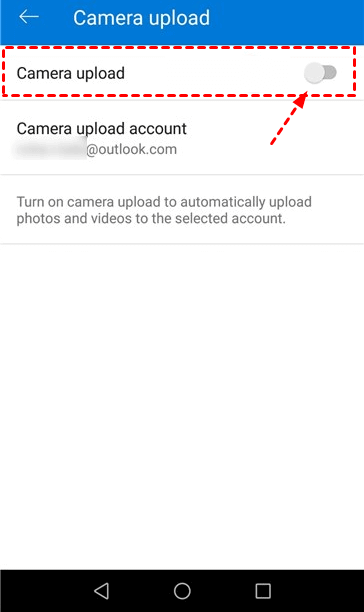A screenshot from a mobile application interface is displayed. At the very top, there's a blue header labeled "Camera Upload" in light gray text. An arrow icon pointing to the left is present within the blue rectangle, likely intended to navigate back to the previous screen.

Below the header, the text "Camera Upload" appears again, accompanied by a toggle switch that can be slid on or off to enable or disable the feature. Further down, a section titled "Camera Upload Account" is visible, but the specific account name is blurred except for the domain "outlook.com."

A description follows, instructing users to turn on Camera Upload to automatically upload photos and videos to the selected account. At the bottom of the screen, a black bar incorporates three icons: a back arrow on the left, a circle in the center (possibly for initiating an action), and a square on the right (likely for stopping the action). The overall layout is minimalistic and functional, providing users with straightforward options to manage their camera uploads.